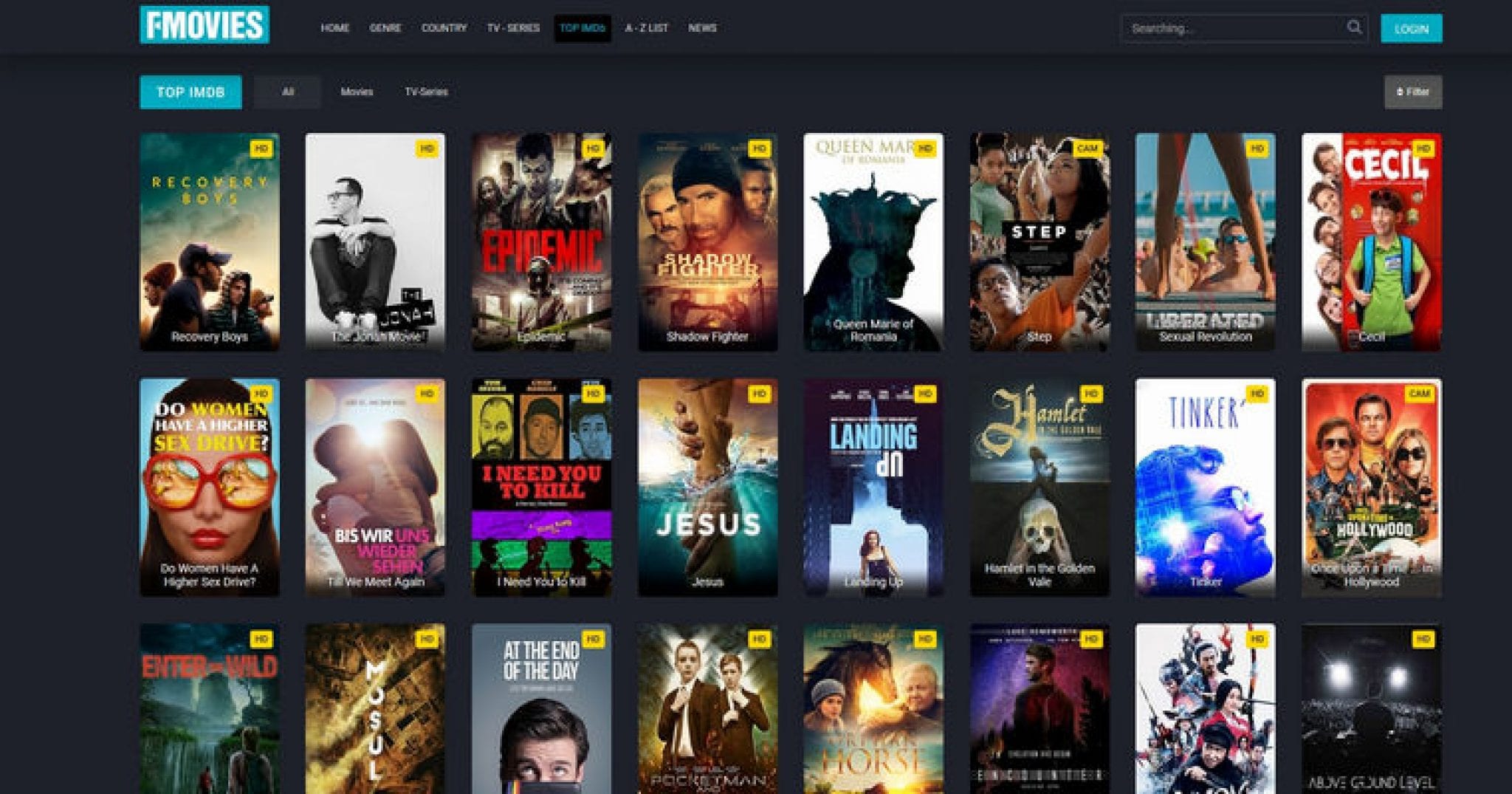This image is a screenshot from a website called fmovies, a platform that allows users to illegally stream films and television shows without a subscription fee. The screenshot appears to be taken from a desktop or laptop displaying a browser window in widescreen dimensions. The website has a dark background, giving it a sleek and modern appearance.

In the top-left corner, there's a blue rectangular box serving as the site’s logo, which features the word "fmovies" in bold, white block letters. Adjacent to the logo, there are multiple navigation links, including 'Home', 'Genre', 'Country', and 'TV Series', allowing users to easily browse through different sections of the site. Beneath these links, there are additional tabs such as 'Top IMDB', 'All Movies', and 'TV Series', offering further filtering options for the content.

The main section of the screenshot displays a grid comprised of eight columns and three rows, showcasing a total of 24 film cover artworks. Each cover is neatly aligned, offering a visual catalog of movies available for streaming. The overall layout is designed to make it easy for users to browse and select the content they wish to watch.